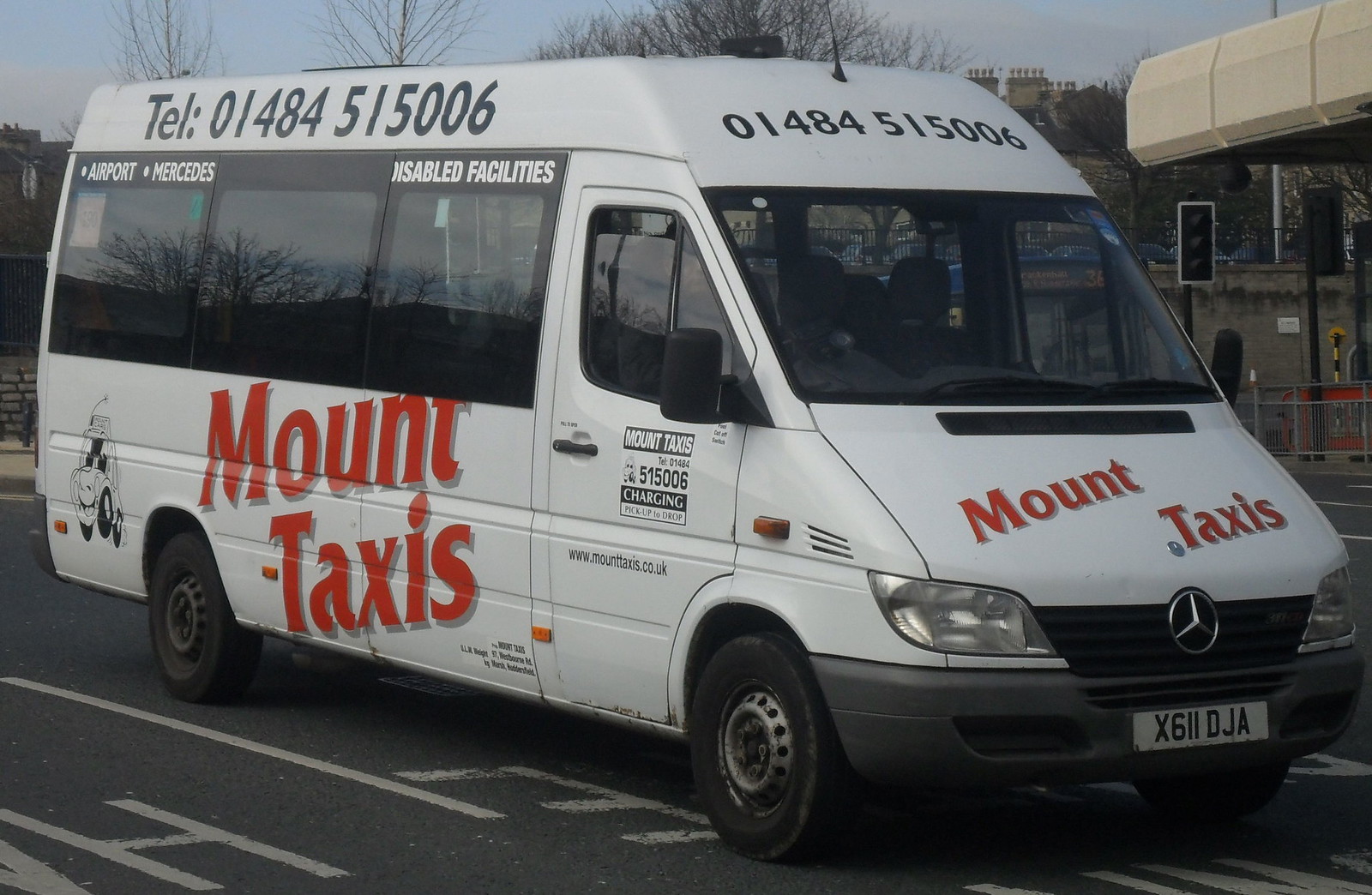The image features a large white Mercedes van prominently branded as "Mount Taxis." The van is parked on what appears to be a black street, possibly a parking lot. The vehicle is adorned with various pieces of text and information. In red font on both the front hood and the sides, it displays "Mount Taxis." The telephone number, 01484 515006, appears repeatedly across the vehicle, including above the windshield in red and alongside the van in black with the prefix "TEL:". The side of the van boasts three windows, and above these, there is crucial information like "Airport," "Disabled Facilities," and illegible text. The front license plate reads X611DJA. Additionally, the side passenger door bears further details about the services offered, spelled out as "Charging, Pick up to drop," alongside the website "www.mounttaxis.co.uk." The repeated mention of various facilities, such as airport transfers and disabled access, underscores the van’s dual role as both a shuttle and taxi service in the U.K.